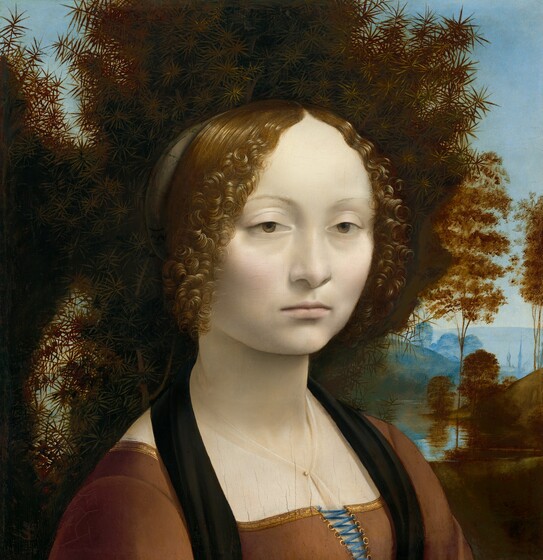This painting, likely from the 16th or 17th century, depicts a dispassionate and youthful woman with pale, porcelain-like skin. Her expression is solemn, and she gazes slightly to the right. Her hair is a reddish-brown, with curly strands framing her face while the rest of her hair falls straight to her shoulders. She wears a brown dress, intricately detailed with blue thread and brown seams tying it together at the chest. The dress features an old-fashioned design, hinting at its historical context. 

Her cheeks and lips are subtly tinted with a very light pink. Surrounding her head, the background shows blurred brownish trees with a pine tree-like bush. Further back, a river or pond reflects the blue sky, adding serene accents to the composition. A landscape of rolling hills and clear blue skies adds depth, creating a harmonious blend of natural and human elements. The meticulous detailing and the overall mood evoke the timeless quality reminiscent of classic masterpieces like the Mona Lisa.